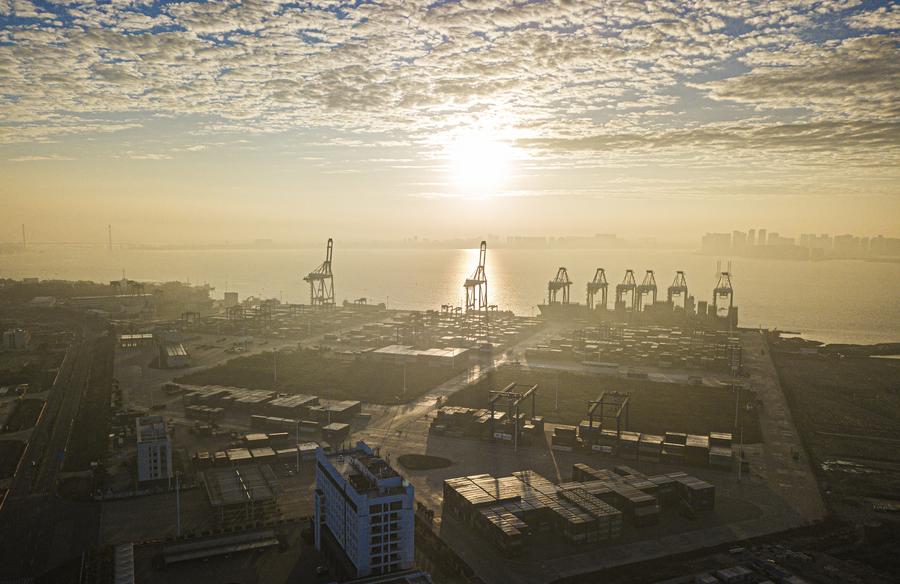This aerial photograph, taken in landscape orientation during the day and pointing towards the sun, captures a bustling port area adjacent to a large city bay. The upper part of the image features a sky partially covered by pillowy, broken clouds with patches of blue. Sunlight streams through the clouds, casting light over the entire scene. On the far horizon, a bridge silhouette appears to the left, set against the outline of numerous skyscrapers.

The central foreground is dominated by a substantial body of water, backed by a series of docks equipped with numerous cranes. Specifically, six to eight large cranes are visible, some actively unloading a ship docked at the port. The ship is laden with cargo containers, many of which are stacked in organized grids on the land behind the cranes. To the right of these cranes, rows of additional containers are scattered across the area.

In front of these stacked containers, closer to the viewer, lies a narrow concrete road flanked by patches of grass. Prominent on the left side of the image is a tall white rectangular building, approximately seven to twelve stories high. Several other white buildings of similar height are positioned around it. The overall scene captures the intricate network of infrastructure supporting the port's operations, with the harmonious interplay of sea, sky, and urban development contributing to the vibrant industrial landscape.